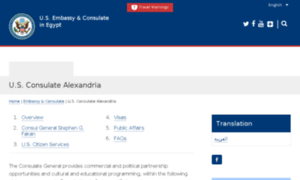A screenshot of a web page is displayed, primarily featuring a white background with a prominent blue banner stretching horizontally across the top. The banner, adorned with the emblem of the United States on the left, showcases a detailed circle containing the frontal view of a bald eagle. The eagle is depicted with a vivid yellow beak, a pristine white head, and rich brown feathers, with the American flag's colors—red, white, and blue—emblazoned in the middle.

To the right of the emblem, written in white text, is the title "U.S. Embassy and Consulate in Egypt." Just below this text, a thin red banner spans across, though the text within it is difficult to decipher. Further to the right, various social media icons—Twitter, Facebook, Instagram, and likely Snapchat—are aligned next to a small magnifying glass icon that indicates a search function.

The body of the page beneath the banner is predominantly white, with black text on the left side reading "U.S. Consulate Alexandria." Following this, the text transitions to blue and provides contact information, including services like public affairs and U.S. citizenship services, catering to inquiries from the public.

Adjacent to this information is another smaller blue banner, with the word "Translation" written in white inside it. At the very bottom of the image, there is a line of small text, though its content is challenging to discern.